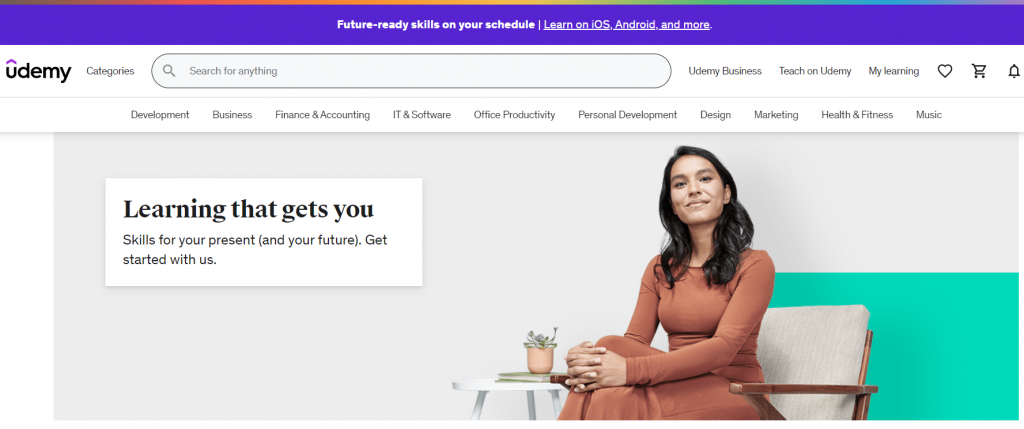In this screenshot, the image features a prominent blue banner at the top, adorned with a colorful rainbow border. The white text on the banner reads: 'Future Ready Skills on Your Schedule. Learn on iOS, Android, and more'. Just below this, a white banner displays the company name 'Udemy' in bold black text. To the right of this, there's a category selection followed by a search bar with the placeholder text 'Search for anything'.

The focal point of the image is a color photo of a young, attractive woman wearing a long brown dress with long sleeves. She is seated comfortably on a beige and wooden chair, looking forward with a pleasant grin. Her arms are crossed over her knees, lending a relaxed yet focused expression. To her left is a small white table, and beside it is a small potted plant housed in a white box with black text. The text reads: 'Learning that gets you skills for your present and your future. Get started with us.' Notably, 'Learning that gets you' is highlighted in bold black text.